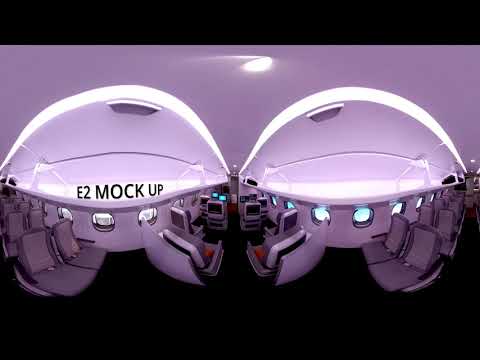The image depicts a highly stylized, panoramic interior view of an airplane cabin, specifically an E2 mockup, as noted by the text "E2 Mock Up" in black letters on the left side of the image. The cabin is split longitudinally, creating a comprehensive view of both sides of the aisle. The seats are arranged in a 2x2 formation and are grey and light grey in color, with small circular windows along the walls indicating this is indeed an aircraft. Each seat is equipped with personal TV screens on the backrests for passenger entertainment. Overhead bins are visible on both sides, and the ceiling lights are turned on, adding to the bright natural daylight streaming through the windows. Despite the detailed furnishings, the cabin is empty of people, emphasizing the mockup nature of the image. The bottom of the image is black, contrasting with a light purple hue at the top, further adding to the surreal and warped perspective created by stitching multiple photos together to form this 360-degree view.